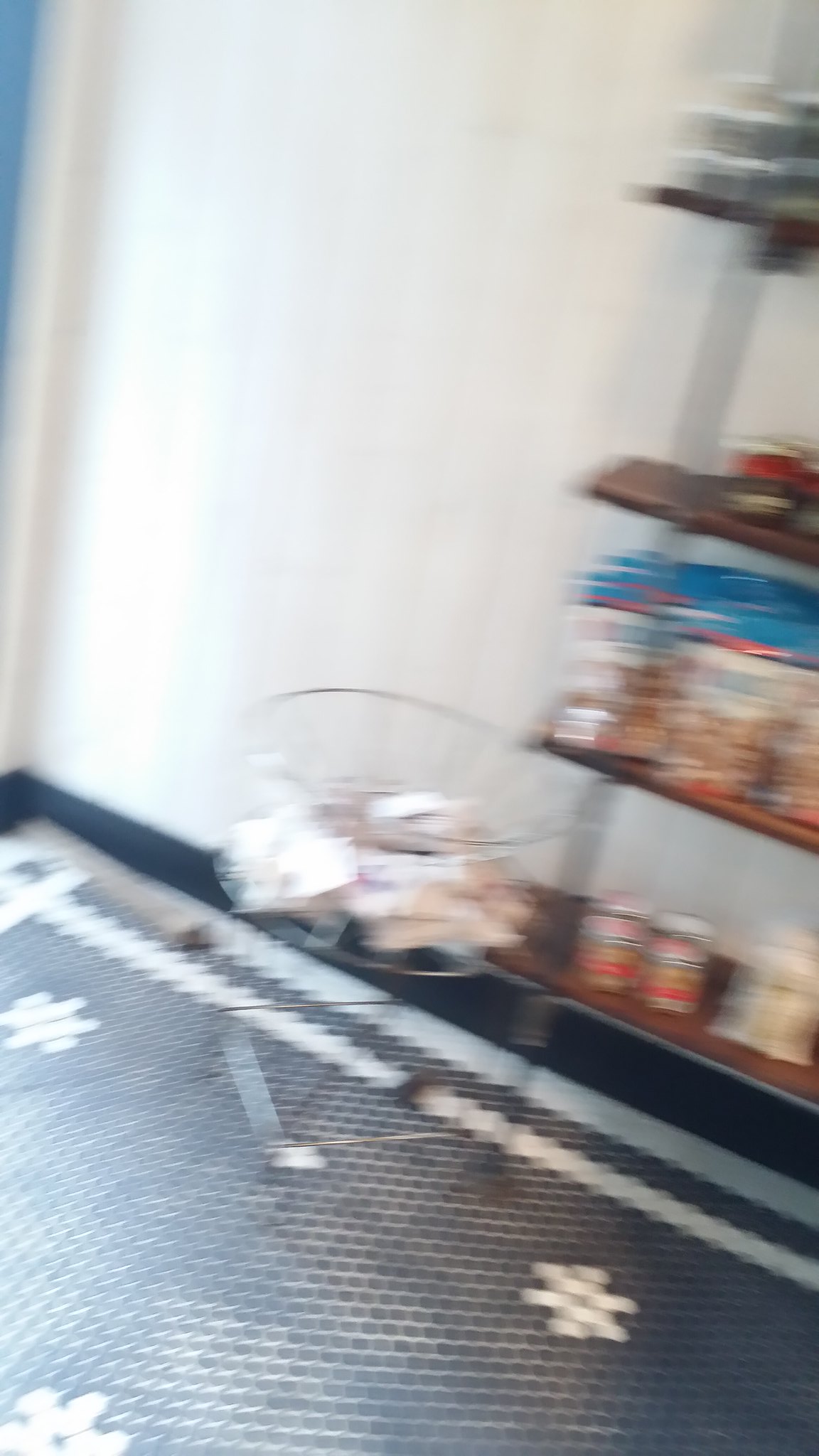This is a somewhat blurry photograph taken from above, showcasing a container filled with white objects, likely dog bones, situated in what appears to be a pet supply store. The primary focus is a white wire container positioned on a matching wire base. In the background to the right, there are shelves stocked with various cans and bags, suggesting an assortment of pet products. The room has a distinctive hexagonal tile floor, patterned in black with white portions and what appear to be white snowflake designs. The walls are painted white with blue trim, and the image captures a corner of the room at the top right, adding to the sense of space.